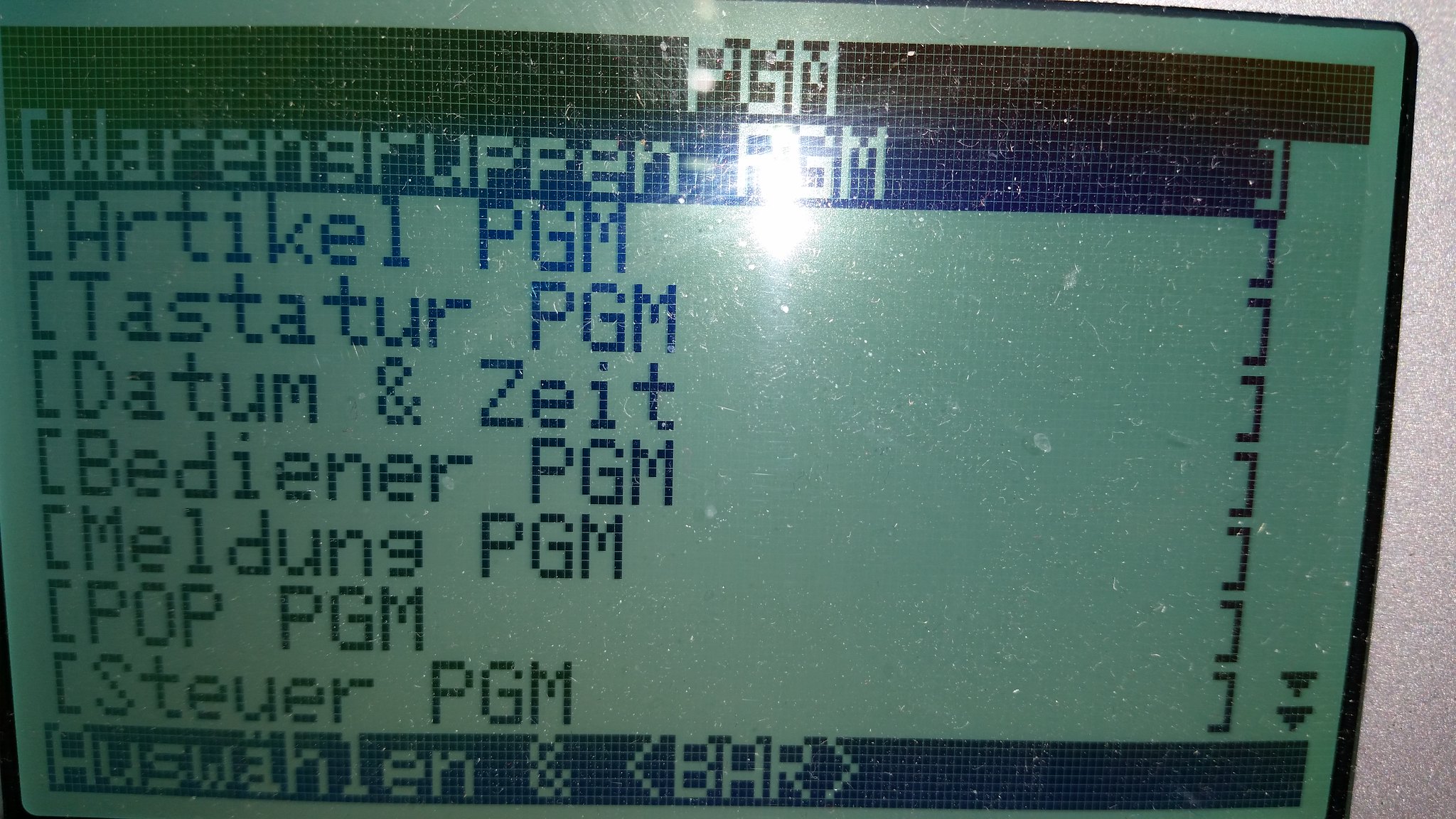The image is a close-up photograph of a low-resolution digital screen with a small display, bordered in silver. The screen displays text in black against a green background. At the top of the screen is the label "PGM," indicating the menu. Below "PGM," there are several menu items listed in what appears to be German: "Warrant Groupen PGM," "Artikel PGM," "Tastatur PGM," "Datum PGM," and "Zeet," which is not followed by "PGM." Lower on the screen, the text reads "Bay Diner, Maldon, Pop, Steyr." At the very bottom, it displays "Ausweilen" and "Bar." The right side of the photograph shows a gray area where the screen ends. The specific device displaying the screen is unclear; it could be a point-of-sale terminal, a control interface, or another type of digital device.